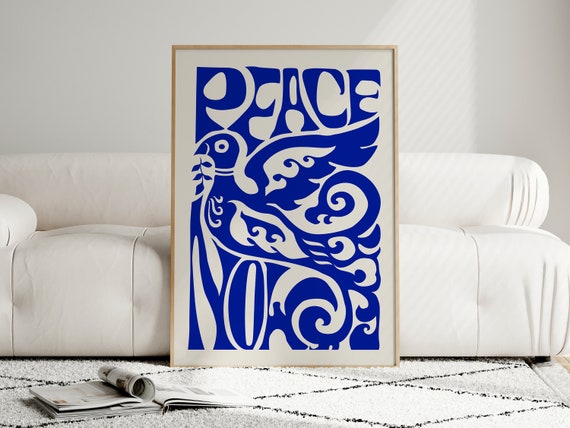In this photo, we see an interior scene featuring a large white couch that stretches across the center from left to right. Positioned prominently in front of the couch is a boldly designed poster in a thin beige frame. The poster, with a white background, features blue, psychedelically-styled letters spelling out "Peace" at the top. Below the text, a blue, dove-like image captures attention, its beak facing left, with a dot for an eye, and its wing extending to the right. The framed poster appears to be about five feet tall and several feet wide. The scene is grounded by a white carpet with a diamond pattern created by black crisscross lines. In the bottom left of the photo, on the carpet, lies an open book or magazine, adding a touch of casual detail to the elegant setting.